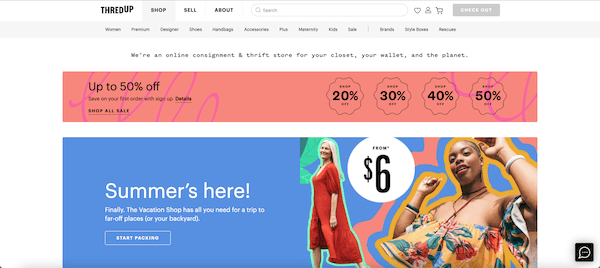This image is a detailed screenshot of the Thread Up website in landscape mode, highlighting various sections and features. 

At the top of the interface, in the upper left corner, are multiple tabs labeled "Thread Up," "Shop," "Sell," and "About." The upper right corner features a subtle button labeled "Check Out." 

Below this, there's a gray navigation bar, although the text is difficult to read distinctly. It appears to include links for categories such as "Women," "Designer," "Shoes," "Handbags," "Accessories," "Plus," "Maternity," and possibly "Kids."

A subsequent row lays out the company's mission statement: "We're an online consignment and thrift store for your closet, your wallet, and the planet." 

The next section advertises significant discounts, stating "Up to 50% off. Save on your first order with..." followed by more details. To the right of these savings, there are clickable buttons displaying various discount percentages of 20%, 30%, 40%, and 50%.

Further down, on a light blue background, the focus shifts to a promotional segment. On the right side of this section, there is a model dressed in an orange outfit and another model in a summery attire. The text to the left states, "From $6," and announces that "Summer's here finally." It promotes "The Vacation Shop" with the caption, "The vacation shop has all you need for a trip to far-off places or your backyard." A clear button labeled "Start packing" invites users to explore more.

This screenshot encapsulates Thread Up’s approachable and cost-effective shopping experience that appeals to budget-conscious customers, exemplified by the user's daughter.